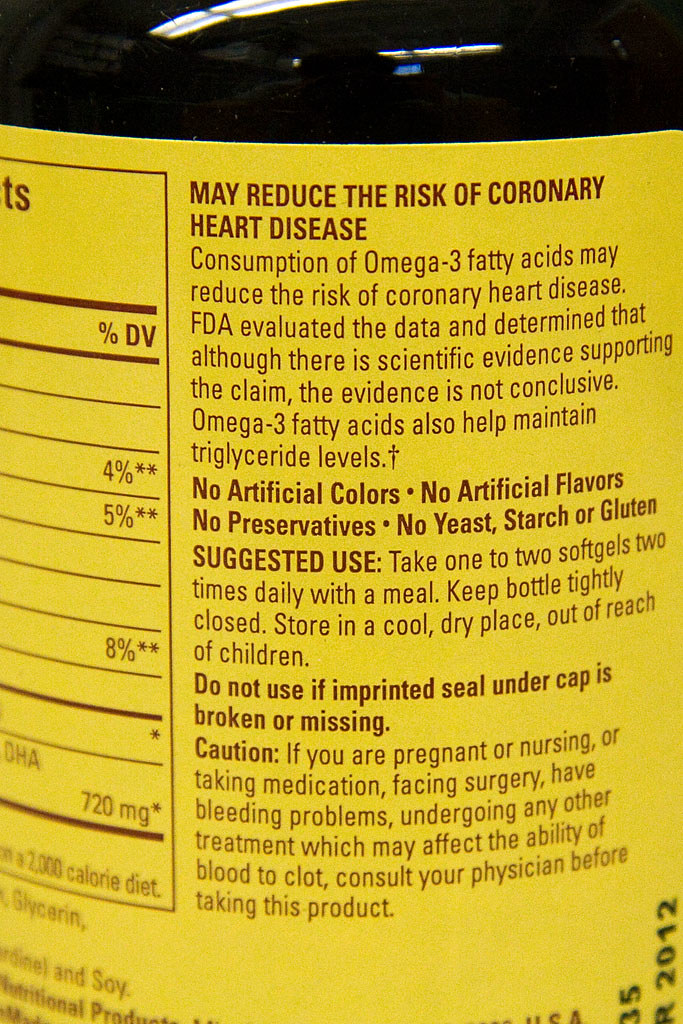This photograph captures a side view of a bottle of medication, focusing on its partially visible label. The label is prominently yellow with dark brown font. A segment of the nutritional facts label is discernible. Notably, the readable portion of the label states:

"May reduce the risk of coronary heart disease. Consumption of omega-3 fatty acids may reduce the risk of coronary heart disease. FDA evaluated the data and determined that although there is scientific evidence supporting the claim, the evidence is not conclusive. Omega-3 fatty acids also help maintain triglyceride levels. No artificial colors, no artificial flavors, no preservatives, no yeast, starch, or gluten. Suggested use: Take one to two soft gels two times daily with a meal. Keep bottle tightly closed. Store in a cool, dry place out of reach of children. Do not use if imprinted seal under cap is broken or missing. Caution: If you're pregnant or nursing or taking medication, facing surgery, have bleeding problems, or are undergoing any treatment which may affect the ability of blood to clot, consult your physician before taking this product."

The bottom of the bottle reveals a partially visible expiration date, indicating the year 2012, though the specific month is unreadable.